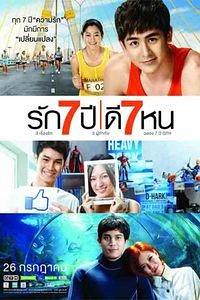This advertisement poster features multiple layered images and text, predominantly in a foreign language. At the top of the poster, a young man with short black hair and a grin, wearing a red tank top, is prominently positioned. Just behind him to the left is a smiling young girl with black hair pulled back, dressed in a yellow tank top with a white strap across the stomach labeled "F-02." In the upper left corner, foreign script appears, and directly beneath it, a white banner reads "S-N-7-U-N-7-K-U," also in the foreign language.

Below this, a second section presents the same young man, now smiling with his teeth visible, and the same young girl holding a white frame in front of her face like she’s looking through glass. A thumbs-up icon commonly seen on social media is placed to their left, with the word "Heavy" visible in the background, suggesting a poster on the wall.

At the bottom of the poster, the background shifts to resemble an aquarium with dark blue water. Here, a different man with dark black hair in a dark blue suit stands beside a woman with red hair leaning against his shoulder, wearing a white jacket with a collar tied around her neck. Overall, the images seem to depict different scenes or moments involving pairs of people in various settings, connected by the advertisement's common theme and foreign language text.